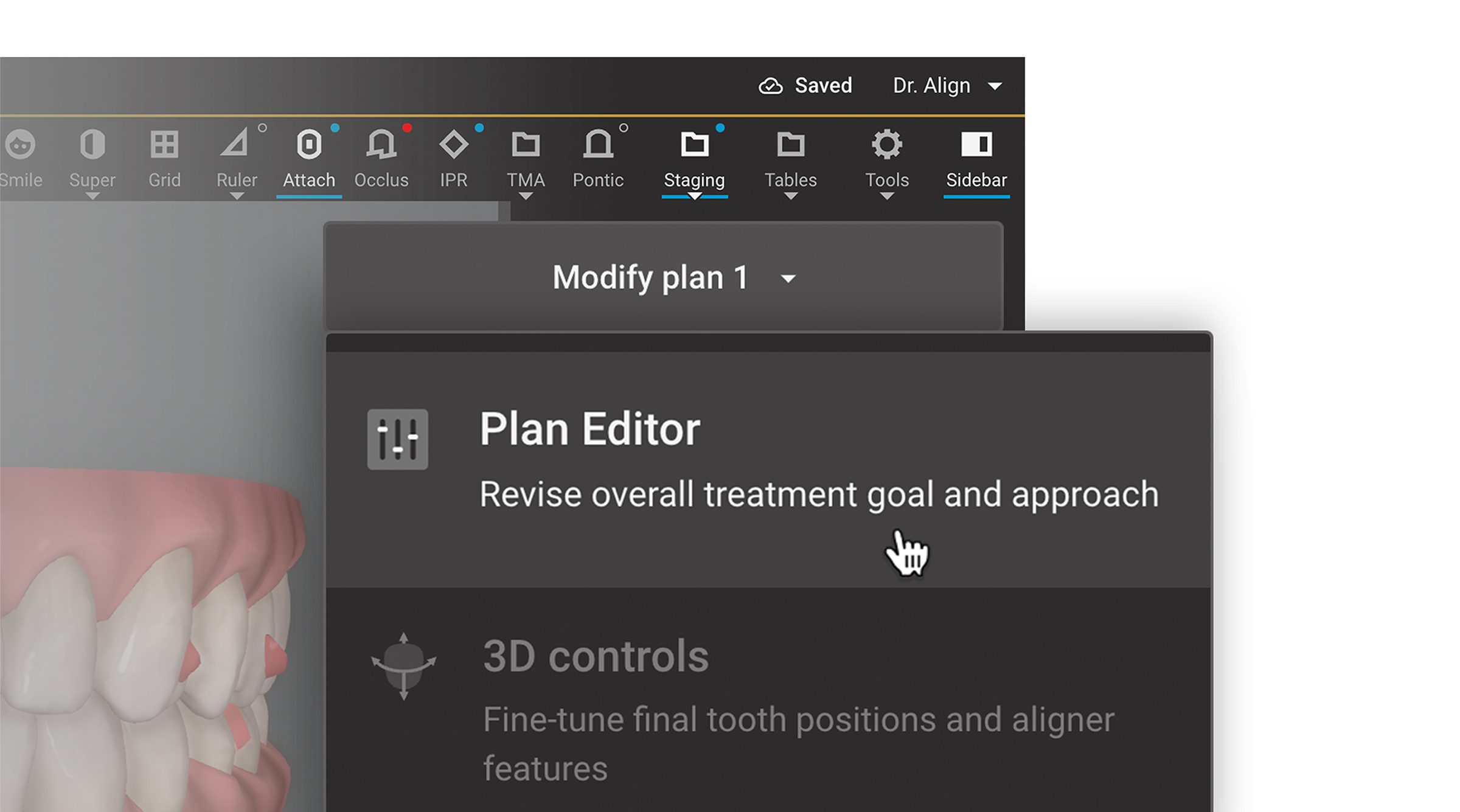The image is a detailed screenshot of dental software with a predominantly dark user interface. On the left side of the screen, partially obscured by pop-up windows, there's a toolbar that includes icons labeled: Smile, Super, Grid, Ruler, Attach, Oculus, IPR, TMA, Pontic, Staging, Tables, Tools, and Sidebar. Towards the middle and right side of the image, there are two pop-up windows. The upper window is a horizontal gray box with white text that reads "Plan Editor: Revise overall treatment goal and approach," with a white gloved hand cursor pointing at it. Below this, there’s a darker gray box that says "3D Controls: Fine-tune final tooth positions and aligner features." Above these pop-ups, there’s a smaller rectangular box that says "Modify Plan One" with a down-pointing arrow. The top bar of the screen features a dropdown menu with a white chevron arrow next to the username "Dr. Align" and a saved icon—a white cloud with a checkmark and the word "Saved" beside it. In the bottom left corner of the screen, there’s a rendering of dentures with pink gums and white teeth.